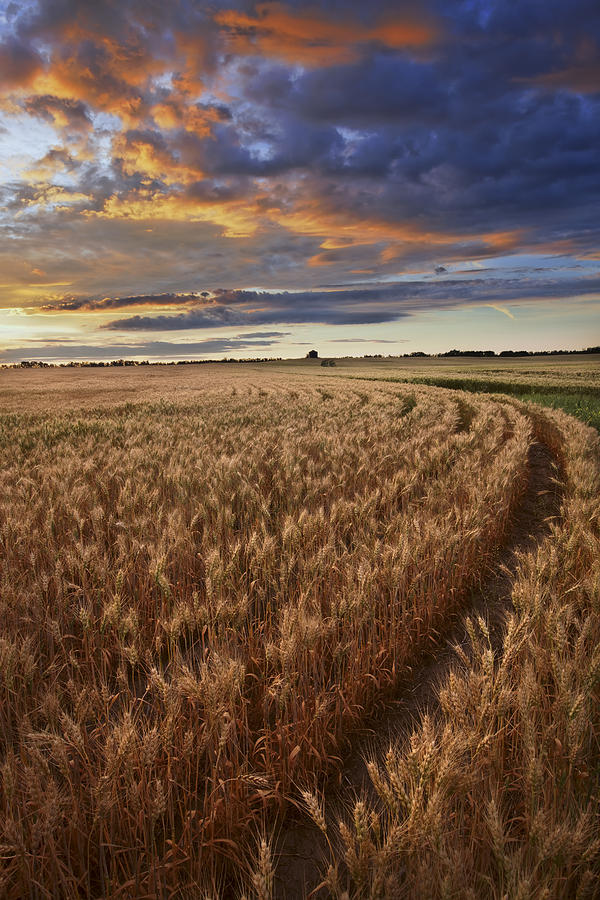This captivating image features a vast, golden wheat field that stretches from the foreground to the horizon, its rich yellowish-brown hues indicating it is ripe or nearing harvest. The field exhibits gentle, undulating curves, notably bending from the right towards the left, with visible rows that seem to both go on infinitely and suggest recent traversal by a sprinkler system or vehicle, highlighted by subtle tire tracks. To the right, there's a patch of green vegetation, its specifics indeterminate, potentially demarcating the transition to more wheat or corn further back. 

The backdrop reveals a distant row of trees and possibly faint structures, nestled against the horizon. Above, the sky commands attention: the bottom third of the image is dominated by this expansive firmament, characterized by a dramatic interplay of colors. Dark clouds interspersed with hues of yellow, orange, and hints of red and purple suggest a sublime sunset scene. The sky’s vivid tones seamlessly complement the earth below, with the darker colors concentrated on the right, blending gradually into the twilight. The striking synergy between the golden field and the painted sky enhances the image's overall aesthetic, creating a mesmerizing, almost surreal visual experience.